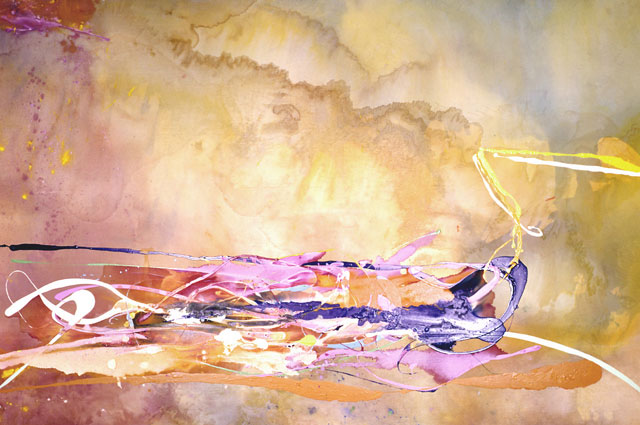This horizontal abstract painting is a whimsical and light-filled composition showcasing a stunning interplay of colors and swirls. The background features a marbleized blend of clouds in soft shades of pink, purple, gold, yellow, white, and blue, creating a dreamy, almost ethereal atmosphere. In the upper left corner, there's a touch of stardust falling through the backdrop, and throughout the upper half, the colors merge into each other, giving a sense of translucency and depth.

Dominating the canvas are ribbons of light and color that weave through the piece in an abstract form, starting from the bottom left and stretching horizontally across without completing the journey. These streaks are vibrant and varied, including hues of pink, orange, yellow, white, and purple, with the occasional hint of burgundy, brown, tan, beige, light blue, and gray. Towards the right side, there's a yellow wand-like shape adding to the whimsical nature of the artwork.

At the bottom, there's a distinct glassy or liquified appearance where orange and blue ribbons look as if they have spilled out and become water. The painting’s overall style is loose, abstract, and rich with beautiful, light-filled colors, creating a scene without specific objects or text, but bursting with movement and imagination.